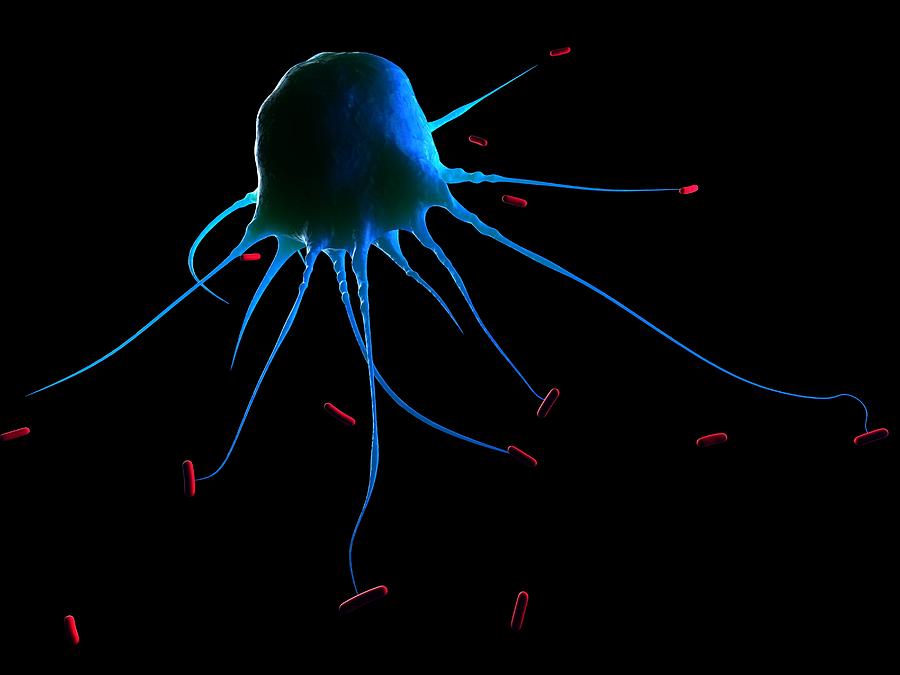This highly stylized and possibly manipulated graphic features a striking jellyfish, illuminated in a glowing blue with hints of green and black, set against a pitch-black background. The jellyfish has approximately 10-11 intricate tentacles, extending outward in various directions, some of which reach towards and grasp dark red capsules or "pills" that float around it. These red capsules are scattered throughout the composition, with some firmly attached to the jellyfish's tendrils and others freely floating nearby. The depiction suggests a light source from behind the jellyfish, contributing to its ethereal, glowing appearance.